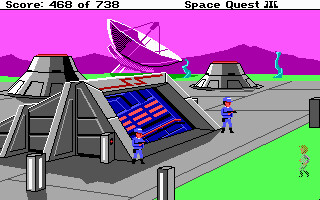A scene from the video game Space Quest 3 is captured in this image. The top left corner displays specific coordinates or reference numbers: 468, 738. The image is pixelated, typical of the era's graphics. Prominently, a radar dish is placed at the top, with cone-like towers positioned on both the left and right sides. The lower right corner features a lush green area where a character appears to be walking or running. In the foreground to the left, a figure is flanked by two guards holding guns, all dressed in blue caps and shirts. The ground is gray, intersected by lines leading to various structures. On the extreme left, there's a tunnel entrance colored in blue, adorned with orange rectangles. Red, squiggly lines can be seen accentuating the top of the tunnel, adding a dynamic element to the scene.